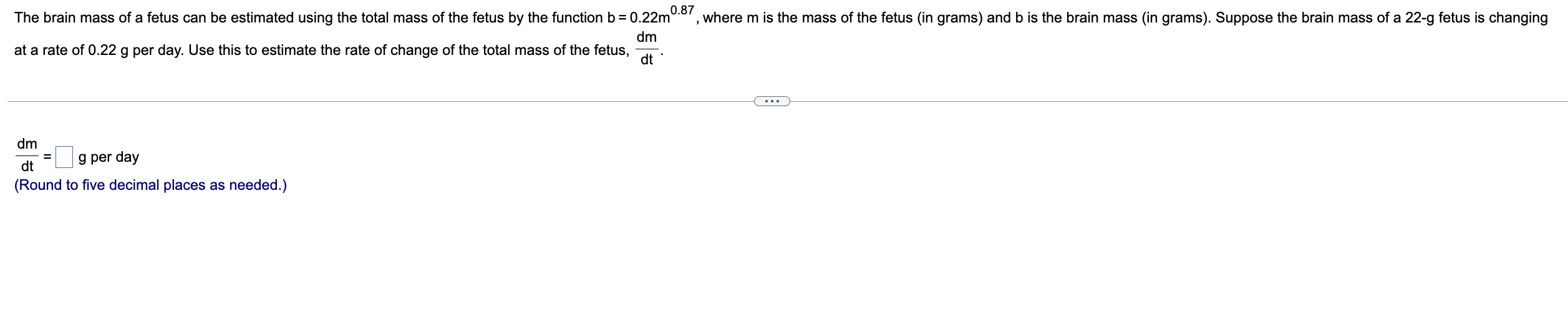**Descriptive Caption:**

The image is a snapshot that appears to be extracted from an educational resource, possibly a biology textbook, focusing on fetal development. The top section of the image contains a mathematical function used to estimate the brain mass (B) of a fetus based on its total mass (M). The function is expressed as \( B = 0.22 \cdot M^{0.87} \), where M represents the mass of the fetus in grams and B represents the brain mass in grams.

The context provided within the image poses a problem that involves a 22-gram fetus, whose brain mass is increasing at a rate of 0.22 grams per day. This data is to be used to estimate the rate of change of the total mass of the fetus, denoted as \( \frac{dM}{dt} \).

Below this problem statement, there is a line with a small oval in the center, enclosing three dotted lines, symbolizing an area for user input or additional information.

Further down, the equation \( \frac{dM}{dt} = \) appears with an empty box designated for the answer, followed by the units "grams per day." In bluish-purple writing, a note in brackets says, "round to five decimal places as needed," providing guidance on the required precision for the answer.

The remaining portion of the image is a blank white space, emphasizing the brevity and focus of the given problem without additional context or distractions.